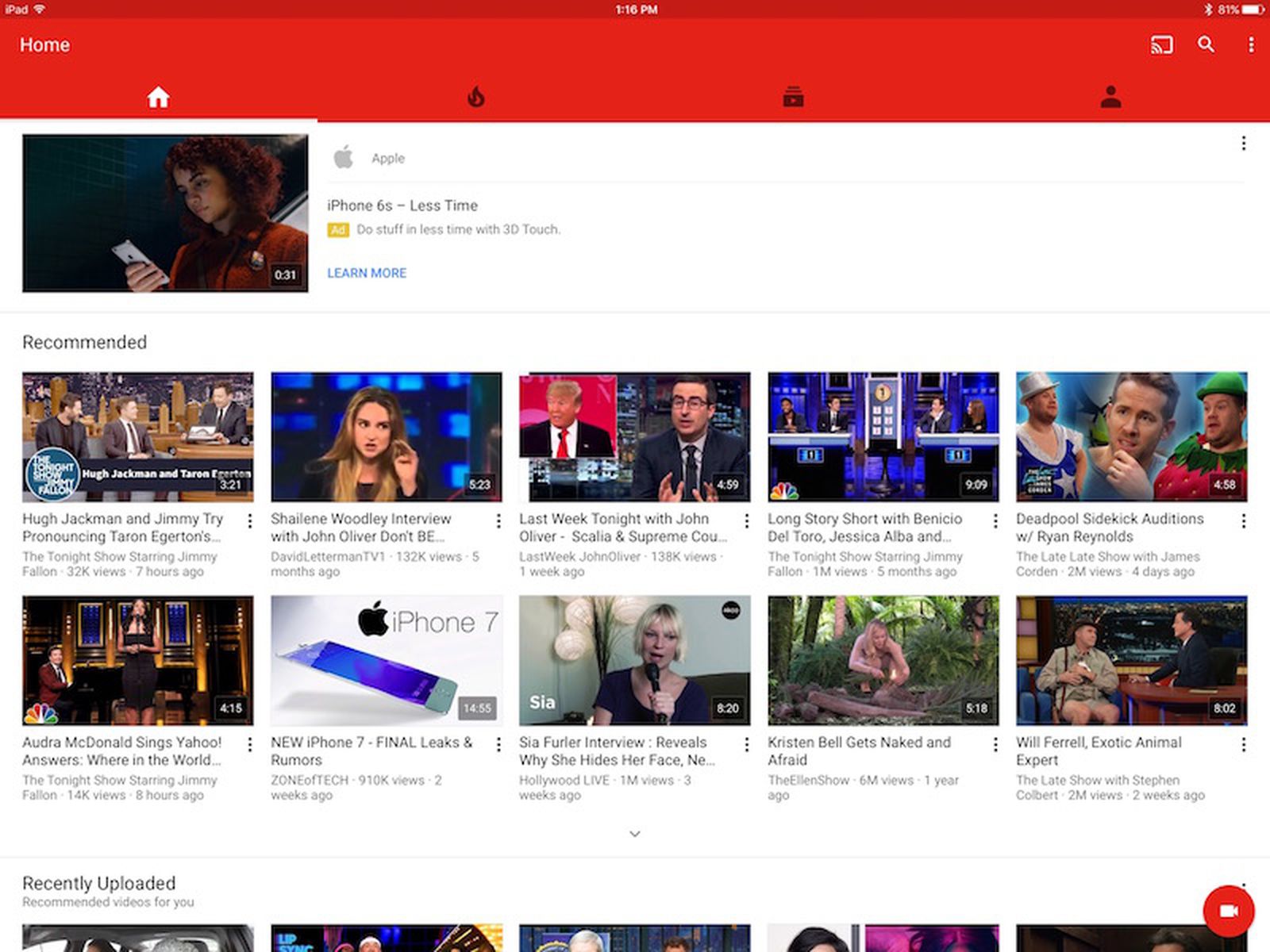This screenshot captures the YouTube app on an iPad, showcasing its layout and several key elements. In the top left corner, the status bar indicates "iPad" alongside a Wi-Fi signal, while the center displays the current time as 1:16 PM, and the far right shows the battery level at 87%. Directly below the status bar is the distinctive red banner of the YouTube app.

On the left side of this banner is a Home icon with the word "Home" beneath it, indicating the main navigation tab. The topmost content visible is an advertisement for the iPhone 6S, featuring a woman engrossed in her iPhone, with the ad duration marked as 31 seconds.

Beneath the advertisement is the "Recommended" section, presenting a variety of ten videos. Among these, notable thumbnails include an iPhone review, a video featuring the artist Sia from Hollywood Live, and a clip titled "Exotic Animal Expert" with Will Ferrell on The Late Show with Stephen Colbert. The layout suggests a diverse selection of content aimed at the user's interests.

At the bottom of the screenshot, partially visible, is the "Recently Uploaded" feed. However, only the top edges of these videos are discernible, making it difficult to identify specific titles or content. The overall interface is consistent with YouTube's design, providing users with navigation options and content recommendations.